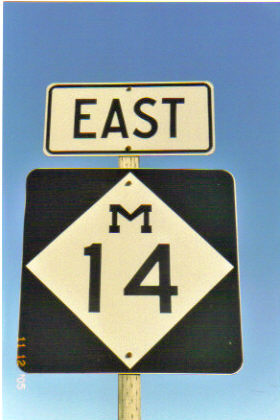In this image, a vertical sign is prominently displayed against a clear sky backdrop. The sign consists of two main sections. The top section is rectangular with a white background and bold black lettering that reads "EAST." Below this, a larger, square section of the sign features a black background with a white diamond in the center. Within the diamond, the black letter "M" is positioned at the top point, and beneath it, the number "14" is displayed in larger text. The sign is mounted on a wooden post, of which only a small portion is visible at the bottom of the image. The post appears to be an artificial, possibly poorly rendered graphic. Additionally, the left corner of the image contains a date in yellow, partially obscured but readable as "11-12," with the text oriented sideways and overlapping slightly onto a blue area.